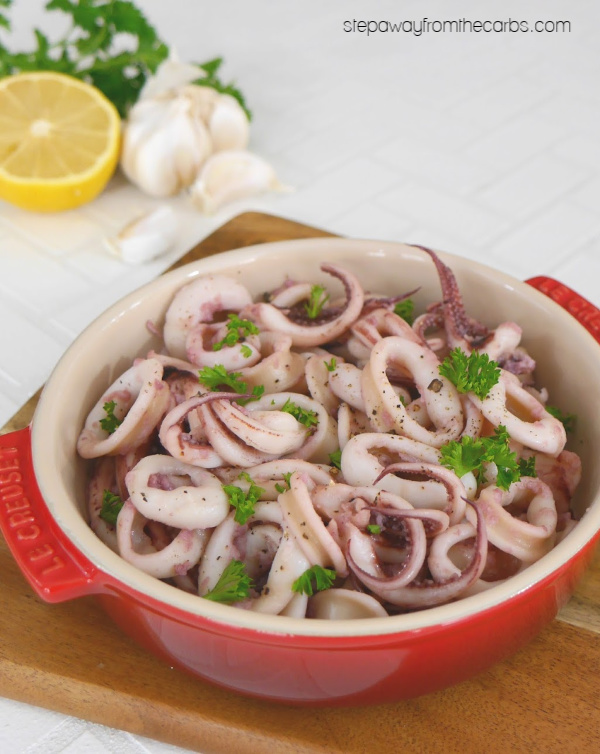The image captures a red enamel baking dish with white interior, placed on a brown wooden cutting board that rests on a white tiled countertop. The baking dish, which features handles with some text on them, is filled with fresh calamari. The calamari, predominantly rings with a few larger pieces and some visible suckers, has been seasoned with green herbs. Off to the side of the dish, on the cutting board, there are sprigs of parsley, a halved yellow lemon, and split garlic cloves. These items also appear slightly blurred in the background of the upper right corner of the image.